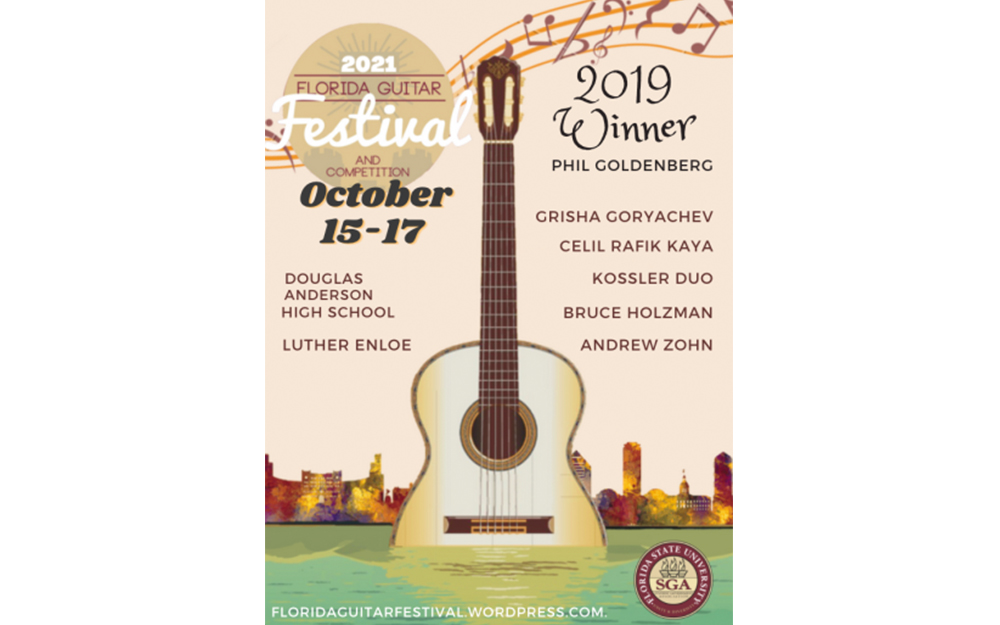The poster showcases the 2021 Florida Guitar Festival and Competition. The image is vertically rectangular with a predominantly pinkish background covering the top 80%. In the upper left corner, a brown circle contains the event title in white lettering, "2021 Florida Guitar Festival and Competition." Below this, in black text, are the dates "October 15-17" and the venue "Douglas Anderson High School." The poster features a design of a single line of musical notes running along the top. Taking up the majority of the space, a large acoustic guitar is partially submerged in water that spans the bottom edge of the image, merging into a multicolored city skyline. Various participant names are listed, including 2019 winner Phil Goldenberg, Grisha Goryachev, Salil Rafiq Kaya, Kostler Duo, Bruce Holzman, Andrew Zahn, and Douglas Anderson High School. In the bottom left, white text reads "floridaguitarfestival.wordpress.com." The lower right corner features the Florida State University logo, a purple circle with a gold seal and the letters "SGA" in the center, surrounded by the text "Florida State University."